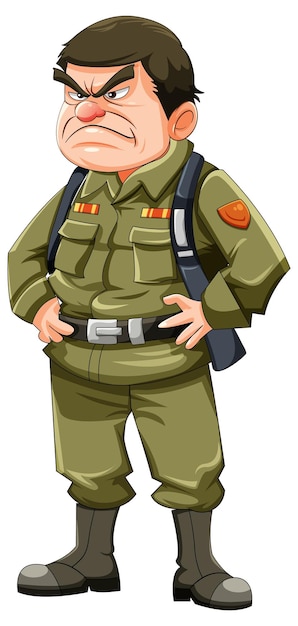This image depicts a cartoon drawing of an older man wearing a green military uniform. His outfit consists of a long-sleeved, button-down green shirt with two chest pockets, each adorned with rectangular red-and-yellow striped badges, and a matching pair of green pants. A black belt with a silver buckle cinches his waist, and the pants are tucked into black boots that reach just above his ankles. A brown shield-shaped patch decorates one of his sleeves, and he appears to be wearing a backpack, as indicated by visible straps. He has a grumpy expression accentuated by thick, inward-pointing eyebrows, a large, round, slightly red nose, and round ears. His hands rest firmly on his hips, adding to his stern demeanor. He also has short brown hair.